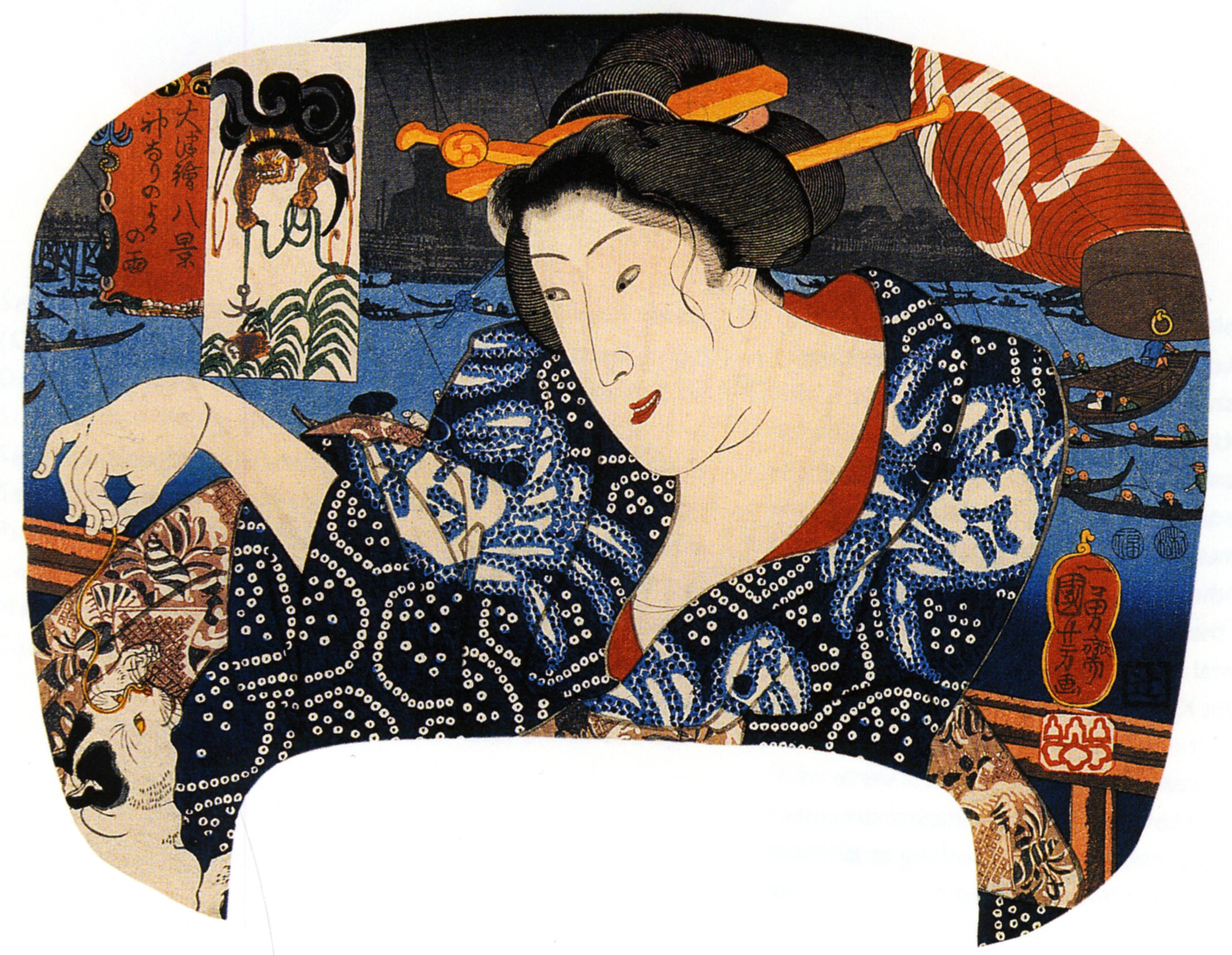The artwork, likely Japanese and from the 1700s or 1800s, depicts a chubby, pale-skinned woman, possibly a geisha, adorned in a beautifully flowing outfit with shades of blue, white, and black, embellished with small white dots and blue-edged flowers. Her hair is elaborately styled into a bun with several ornamental sticks and a hairdresser protruding from it, including one stick possibly holding a lantern. The woman, who has an expression of happiness, is looking off to the left with thin eyebrows, slanted eyes, and a stylized, elongated face typical of Japanese paintings from that era. She holds a piece of thread in her extended hand, playing with a cat at her feet. The background is colorful with a predominantly black base, featuring various elements like a body of water depicted in blue, long narrow boats or canoes with people in them, and a railing behind her. Above her to the left, banners with Asian characters fly, and to the top right of the scene is a red globe-like lantern adorned with white decorations.